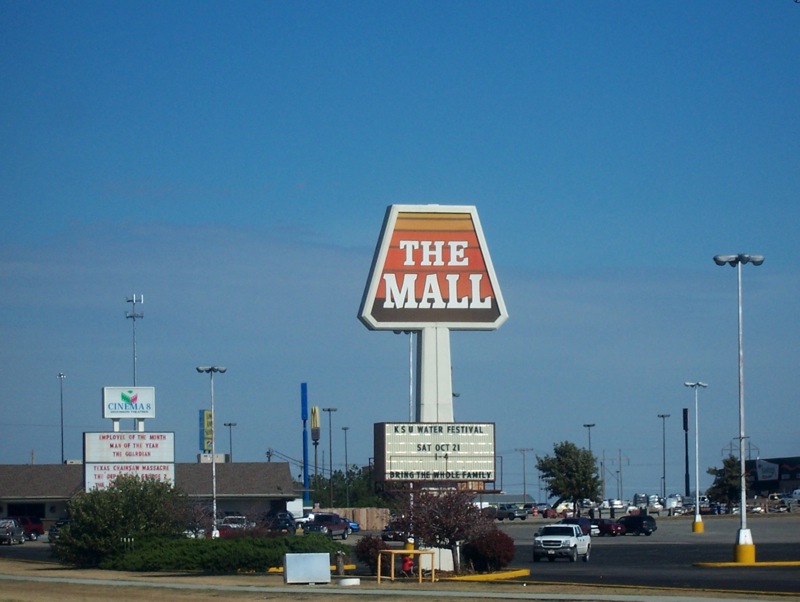The image depicts a bustling street corner adjacent to a sizable parking lot beside a shopping mall. On closer inspection, the area initially perceived as an intersection reveals itself to be the expansive parking area of the mall. Prominently placed at the boundary of the parking lot and the street is a tall sign, which showcases the mall's name in white text against a vibrant, striped backdrop composed of yellow, orange, and brown hues. Ahead in the frame, several tall light posts can be observed, providing illumination for the surrounding area. Numerous cars are parked to the right and throughout the mall's parking space, indicating a busy day. Additional signage is visible, including a distinct blue sign on the left side pointing towards a cinema, enhancing the scene's lively, commercial atmosphere.